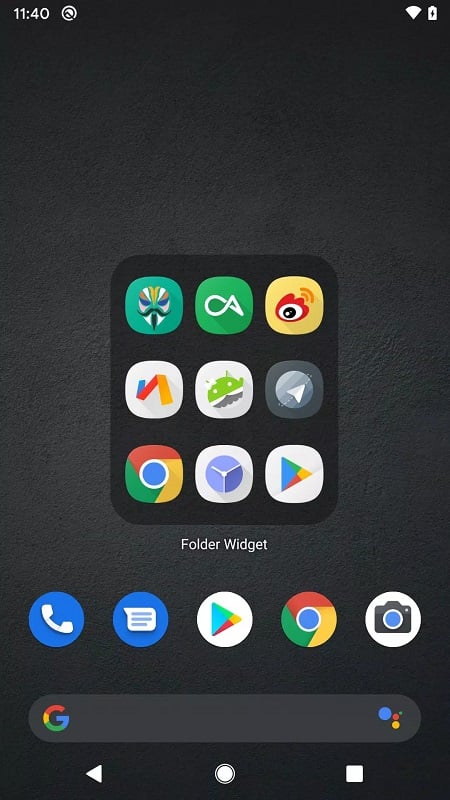**Detailed Caption:**

In this image, we have a smartphone interface displayed against a black background. At the top of the screen, the status bar shows the time as 11:40, with the battery at 100% and full internet connectivity indicated. Central to the display, there is a series of folder widgets encapsulated within a black square box.

Within this folder, there are nine distinct, albeit somewhat unidentifiable, widget icons. Among them, the Google Play Store icon is located at the bottom right, and the Google Chrome icon is positioned on the bottom left.

Below this folder, there are five key app icons arranged horizontally which include: a phone icon, a messaging icon, another Play Store icon (circular), the Google Chrome icon, and a camera icon.

At the very bottom, a gray search bar is prominently featured, adorned with a Google "G" logo to the left side, facilitating quick search access.